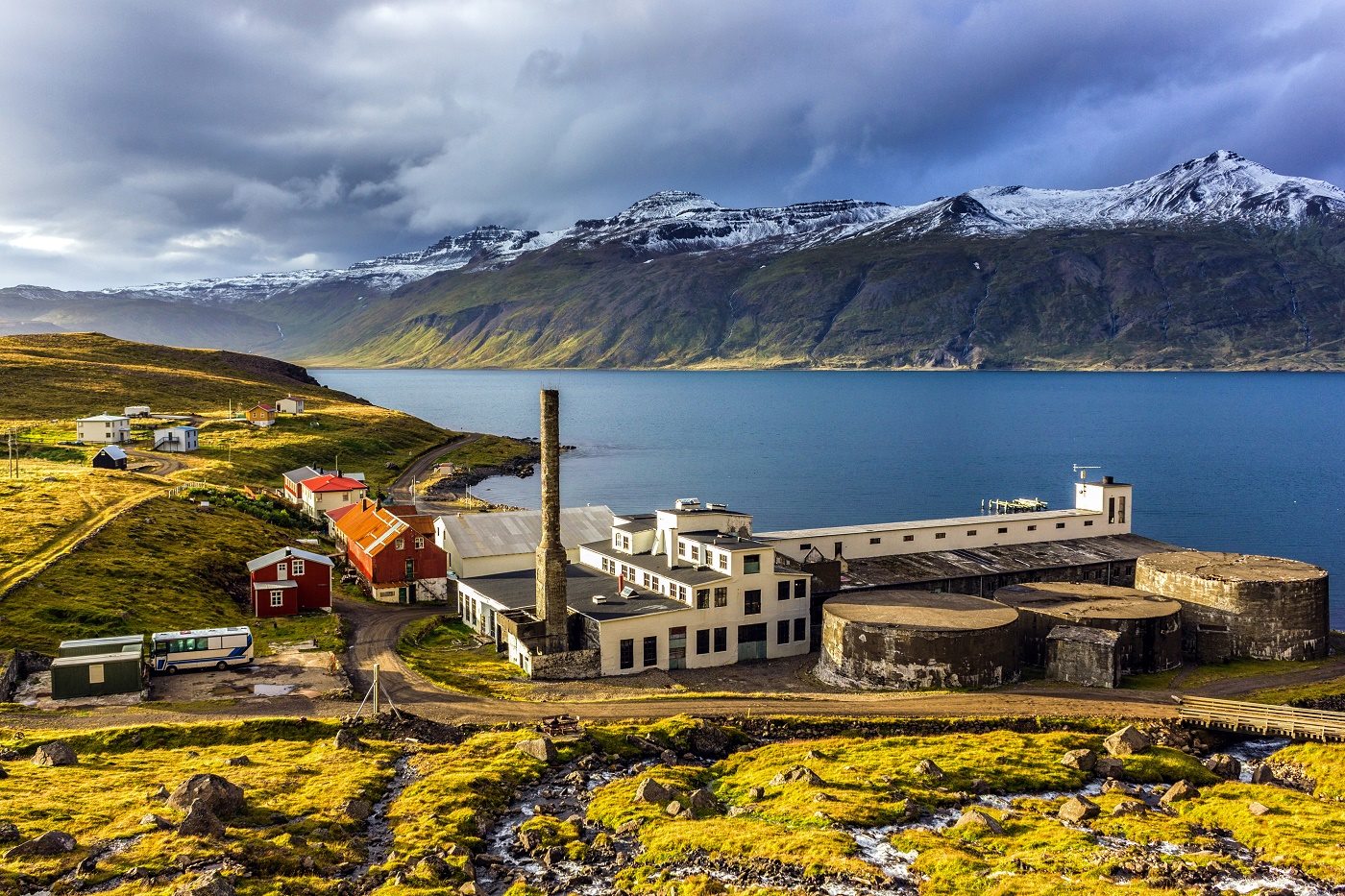This photograph captures a serene lake flanked by lush greenery and rugged terrain with moss and greenish-yellow vegetation. On the right-hand side, the calm, beautiful blue water reflects the dramatic sky, which is filled with gray and white clouds. The backdrop features a stunning range of snow-capped mountains extending toward the sky, adding depth and grandeur to the scene.

In the foreground, a green marshland stretches out, intersected by a dirt road that runs horizontally across the image. Nestled within this marshland is a small, sparsely populated area dotted with colorful structures. A prominent white industrial building with a flat roof and a large cement smokestack stands out. Nearby, various homes, including a red farmhouse with a white roof, a trailer, and a bus, add splashes of red and tangerine to the otherwise muted landscape. Additional round wooden structures, possibly containers, add to the rustic charm.

The whole setting suggests a possibly European location, reminiscent of picturesque Dutch or Scottish landscapes, though it could easily be mistaken for a serene, less-known spot in America. The scene is a harmonious blend of natural and man-made elements, creating a captivating and idyllic panorama.